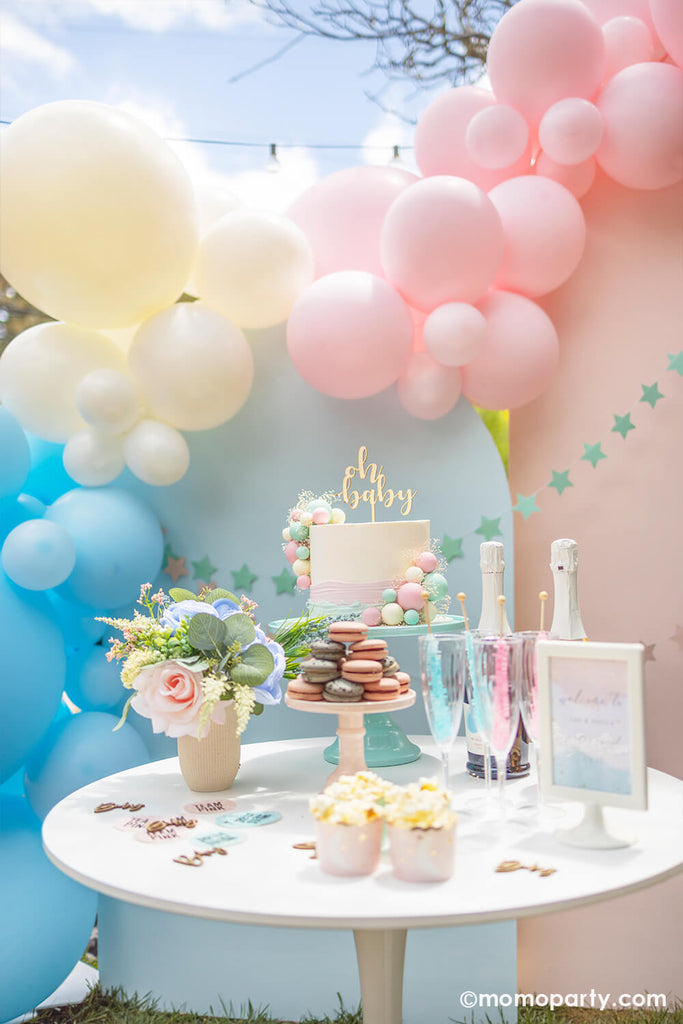This vibrant photo captures a baby shower celebration set against a backdrop of blue sky with wisps of clouds and a distant tree, adorned with hanging lights. The focal point includes clusters of pastel pink, blue, and white balloons, interspersed with blue stars hanging in a line, creating a festive atmosphere. Below the balloons, the scene features large pink and blue boards. Dominating the foreground is a white round table elegantly decorated with a white cake that says "Baby" on top, adorned with multi-pastel colored spheres in pink, yellow, and blue. Surrounding the cake are a vase filled with colorful pink and blue flowers, macaron cookies in a cake holder, two champagne bottles, champagne glasses, and a small white sign advertising the party. On the left side of the table are also noticed strands of rock candy, adding a playful touch to the setup.